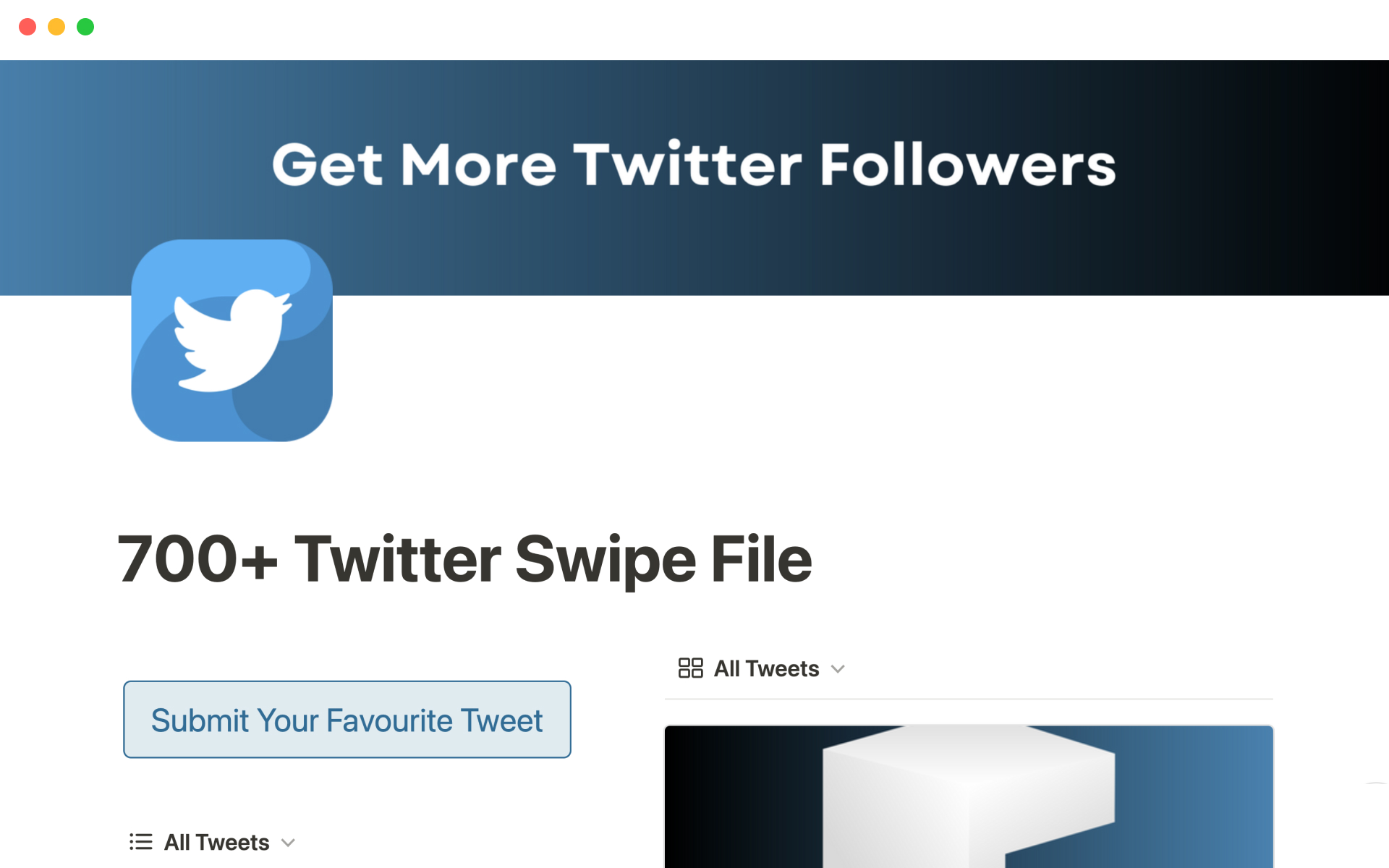The image is a highly detailed, enlarged screenshot from Twitter, or what used to be Twitter before its rebranding to X. The image is in landscape orientation. The bottom two-thirds of the image is predominantly white, while the top portion features a gradient bar transitioning from blue on the left to black on the right. 

Centered within this bar, in large white letters, is the phrase "Get More Twitter Followers." In the top left corner of the white background, there are three small dots in a horizontal row: the first dot is red or orange, the second is yellow, and the third is green.

Below the "Get More Twitter Followers" banner is the iconic Twitter logo, a blue box with a white bird silhouette in the center. Further down, also on the white background, is the text "700+ Twitter swipe file" in blue letters. There is a light blue oblong outline enclosing a dark blue button, which has the phrase "Submit Your Favourite Tweet," with the British English spelling of "Favourite" indicating a UK or similar English-speaking region.

On the right side of the screen, there is a menu icon labeled "All Tweets" accompanied by a dropdown arrow. This menu icon is followed by a graphic consisting of blue, black, and white cubes. Additionally, in the bottom left corner of the image, there is another menu icon also labeled "All Tweets" with a dropdown arrow.